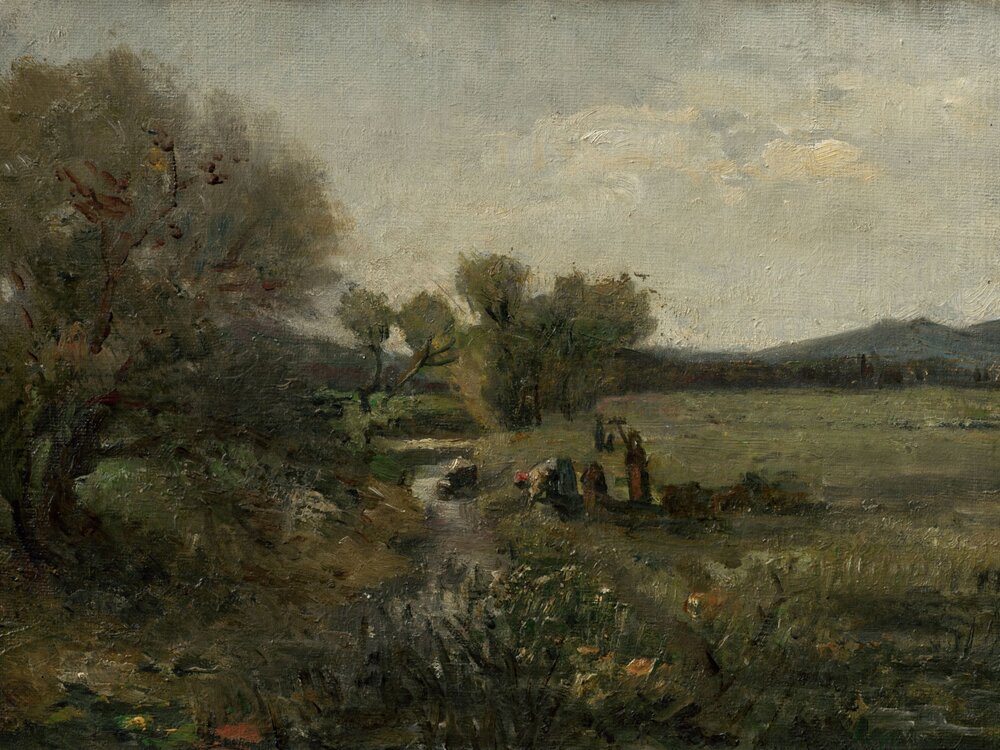This abstract painting captures a pastoral scene by a riverside or small creek that runs through the center of a vast green pasture, possibly an orchard, field, or garden. To the left side of the image, a large tree is prominently featured, surrounded by bushes and other trees, creating a dense background of flora. The right side of the painting opens to a clearer view of the field with green grass. Three people are depicted in the scene, seemingly engaged in some form of activity near the creek. One individual, a woman in a headscarf and dress, is notably bent over as if picking something up from the ground, while another figure stands nearby, possibly assisting or observing. The distant background reveals gentle hills or a mountain under a predominantly gray, cloudy sky with hints of white and faint touches of bright orange. Wildflowers dot the landscape, adding a touch of vibrancy to this otherwise muted, yet evocative, pastoral setting.